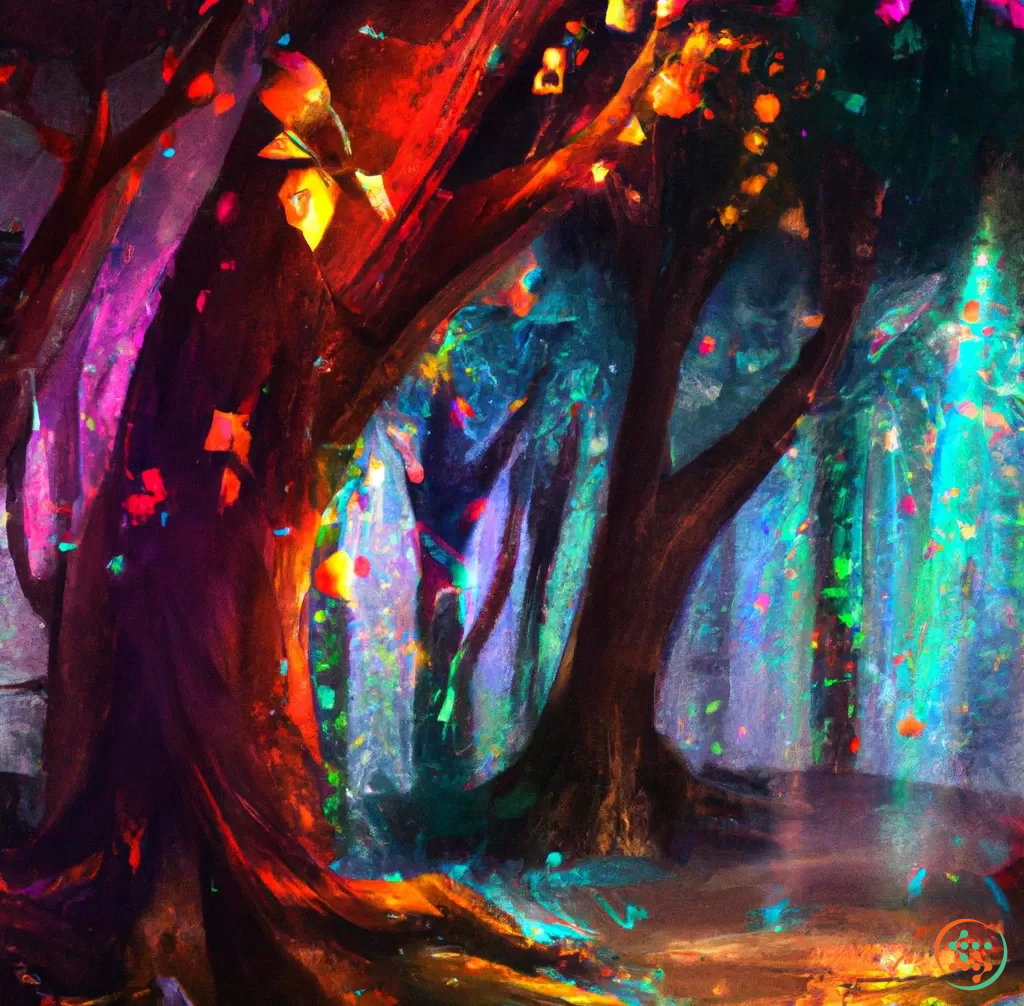This detailed painting, likely an impressionistic watercolor piece, depicts an enchanting fantasy forest scene brimming with vibrant colors and ethereal charm. Dominating the foreground is a large tree with a reddish-brown trunk that wraps around itself, ascending dramatically. This tree features branches adorned with golden yellow leaves that glitter like sparks of light. Surrounding it are other distinctively colored trees, including an orange and brown tree with hints of yellow, a blue tree with pink and yellow accents, and a brown tree with green on its trunk. The forest floor is a rich brown, interspersed with whimsical blue squiggles. The background is awash with a harmonious blend of turquoise, light purples, and blues, creating an otherworldly atmosphere as sunlight filters through, casting an illuminating glow upon the scene. Adding to the mystical feel, a unique symbol, a circle enclosing several dots, is positioned at the bottom right of the painting. Amidst the vivid canvas, there are no text elements, allowing the artwork's colors and composition to convey its dreamlike essence.